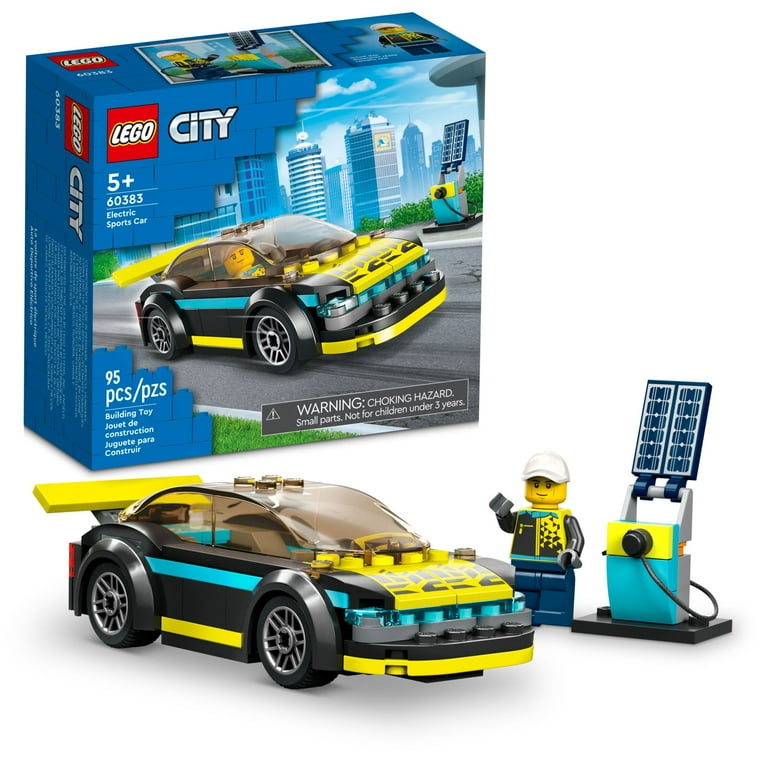This image features a detailed product advertisement for a Lego set. In the upper left corner of the picture, there is a box displaying the Lego logo, a red square outlined in black with "Lego" written in white, and "City" written in silver beneath it. The box details include the set number 60383, labeled "Electric Sports," and indicates it is suitable for ages 5 and older, containing 95 pieces. The front of the box shows an image of the assembled sports car the set can make. The car itself is prominently displayed below the box within the image. This car is distinctive with black sides, a yellow trunk and rear tail fin, along with blue and yellow stripes near the bottom. Next to the car stands a Lego figure, presumably the driver, clad in matching light blue attire. Adjacent to the figure is an electric charging station, also light blue, featuring a yellow square and a black nozzle. This station is topped with solar panels, reinforcing its eco-friendly theme.